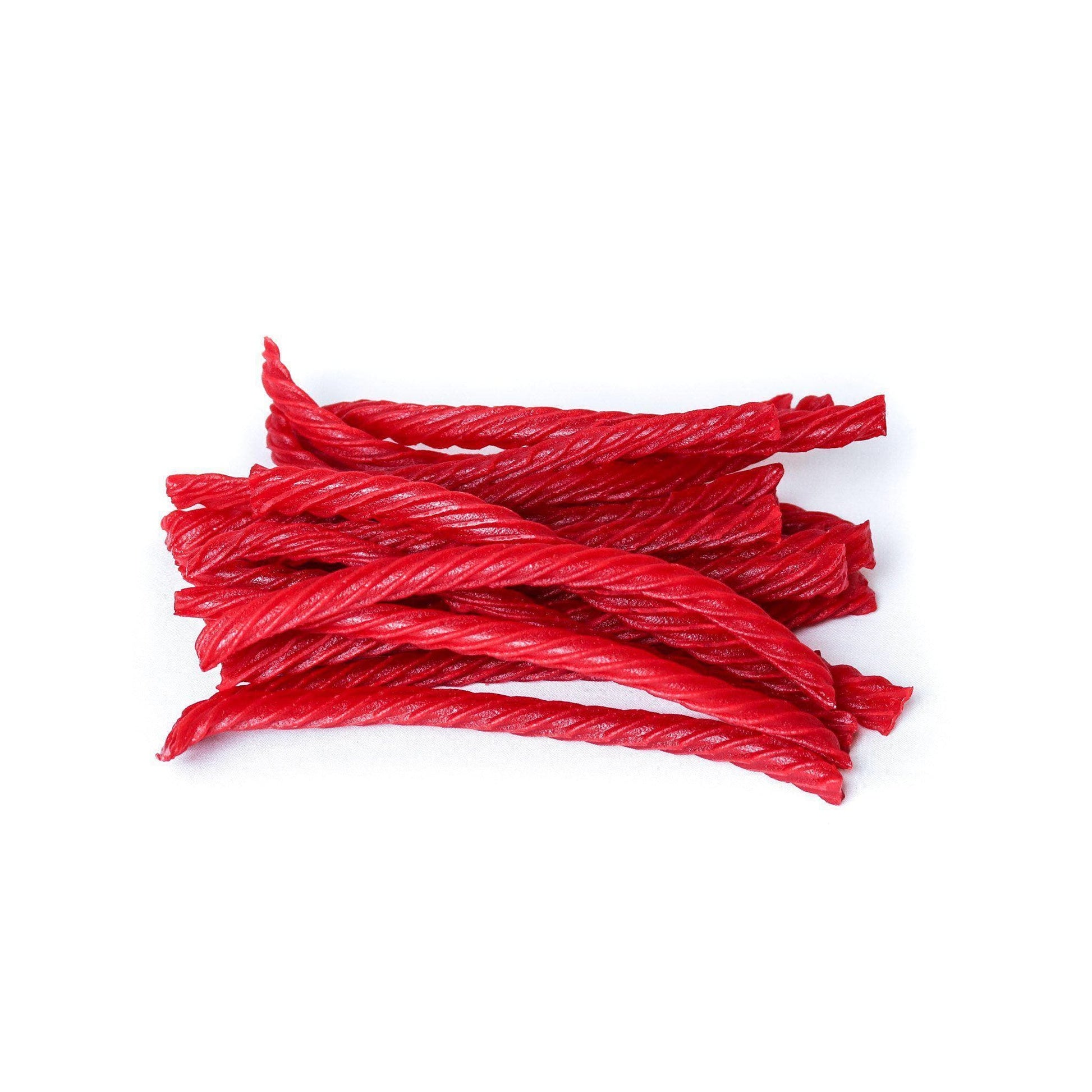The image features an array of twisted, red licorice deeply resembling Twizzlers. The licorice is stacked haphazardly atop one another, with each piece showcasing the typical twist pattern and a manufactured appearance. The vibrant red color exhibits slight variations in shade due to the lighting, casting highlights and shadows that emphasize their glossy texture. The licorice pieces extend horizontally from left to right on a stark white background, enhancing their bold hue. The pile, consisting of approximately 15-20 uneaten pieces, fills the frame, creating dynamic curves and overlaps with occasional white spaces between them. The white background appears clean and uninterrupted, making the red licorice the unmistakable focal point of the image.